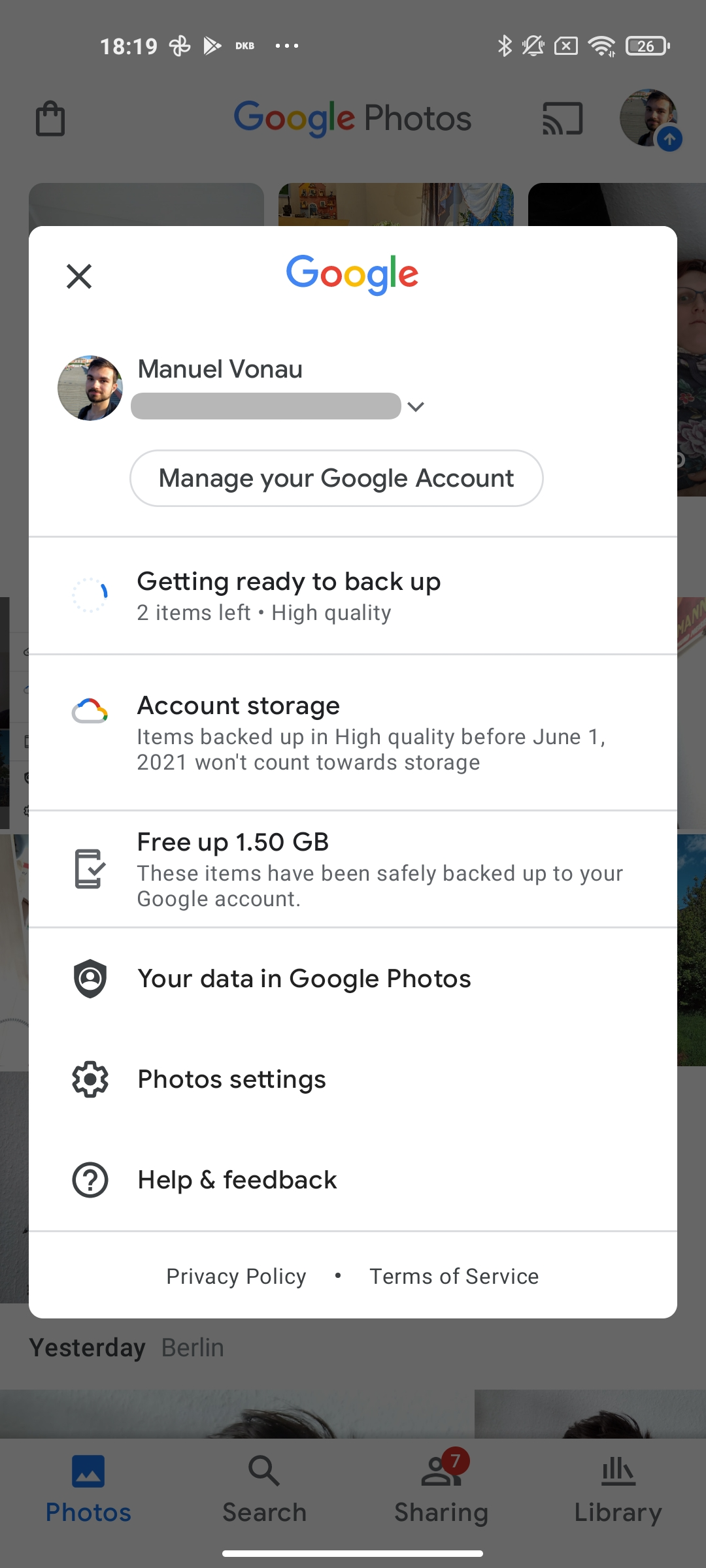At the very top of the image, the time "18:19" is displayed, followed by a small white arrow pointing to the right. To the side, there is a battery symbol with "25" inside it. Below this, there's a long white rectangle with an "X" in the upper corner.

To the right of this rectangle is the word "Google," with each letter colored differently: blue, red, yellow, blue again for the second "G," green for the "L," and red for the "E." 

Underneath this is a profile picture in a circle, showing a man with black hair, labeled "Manuel Vonau." Below this, there is a gray rectangle with several options listed inside ovals: "Manage your Google account," "Getting ready to backup," "Account storage," "Free up to 1.50 GB," and "Your data in Google Photos."

At the bottom, there is a settings wheel icon next to the text "Photo settings," followed by a question mark inside of a circle with the option "Help and feedback" beside it. The very bottom of the image features choices for navigation: "Photos," "Search," "Sharing" (highlighted with a red circle), and "Library."